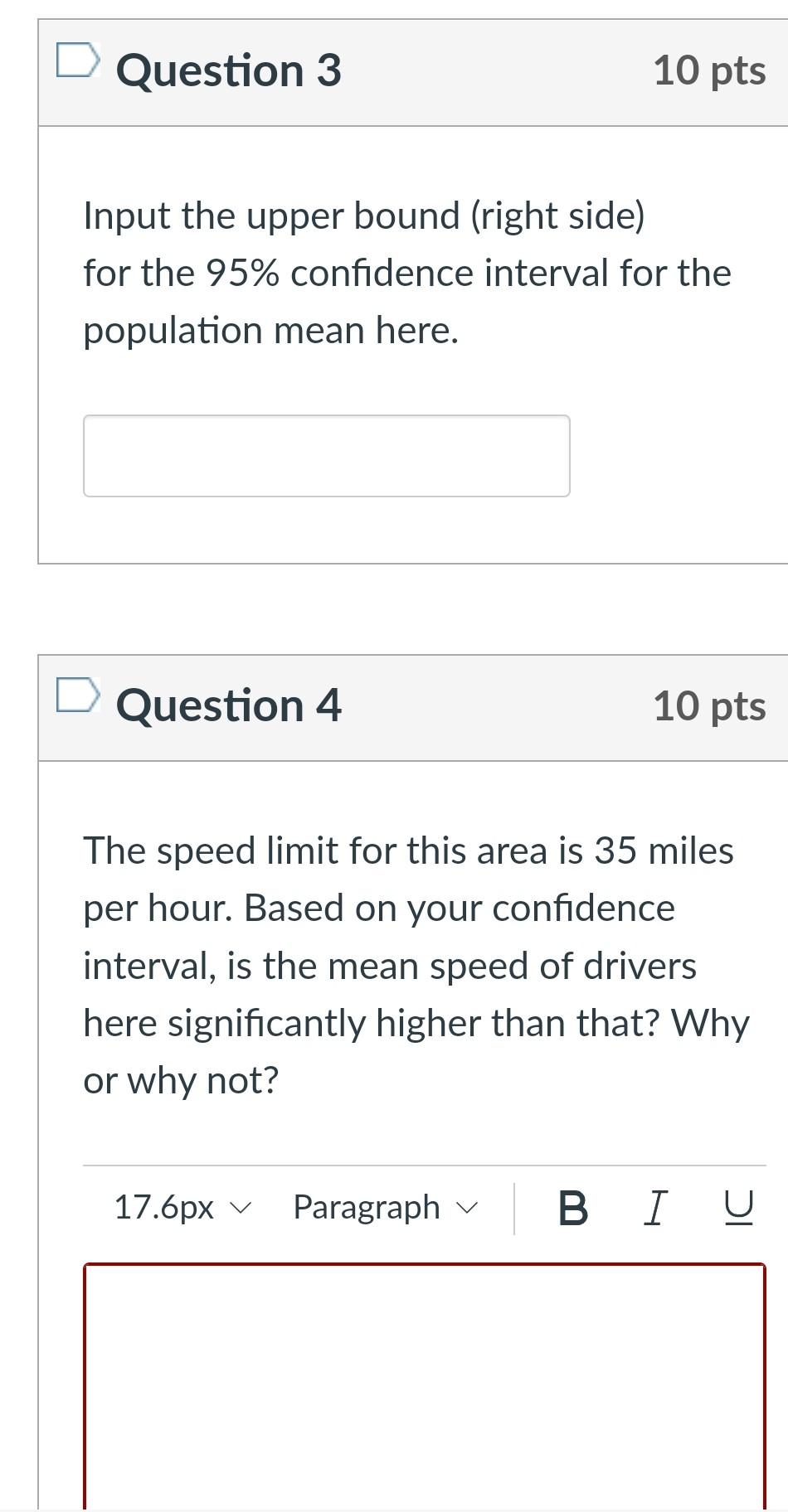The image is a screenshot of a website displaying a series of questions related to statistics. In the top left corner, there's a header indicating "Question 3: 10 points." The prompt for this question reads, "Input the upper bound right-side for the 95% confidence interval for the population mean here," followed by a field where users can enter their response.

Directly below, another section is titled "Question 4: 10 points." The prompt for this question states: "The speed limit for this area is 35 miles per hour. Based on your confidence interval, is the mean speed of drivers here significantly higher than that? Why or why not?" There is a 17.6 px paragraph in bold, italics, and underline formatting. Below this, there is another field designated for users to enter their paragraph response.

This image appears to capture an online statistical assessment, highlighting the questions and spaces provided for user input.